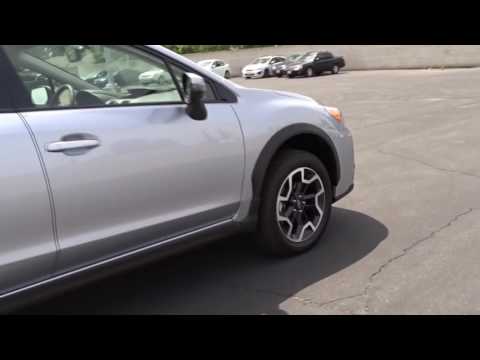The image captures a detailed scene of a parking lot featuring a prominently positioned four-door silver sedan with black wheels and silver rims, located towards the left-hand side of the frame. The car's passenger side is clearly visible, revealing the door, tire, rear-view mirror, and a portion of the window, cropped midway. This silver vehicle is situated on a heavily cracked, light gray asphalt surface without distinct parking spot lines. Extending towards the top of the image, multiple parked cars can be seen in the distance, specifically a black car, a blue car, three white cars, and another black car, all aligned against a concrete or cement wall. Behind this wall, there is lush greenery with trees and vegetation. It appears to be midday, inferred from the short shadow cast by the silver car towards the front of the image, indicating the sun is high in the sky. The setting is outdoors, providing a natural backdrop and casting natural light across the entire scene.